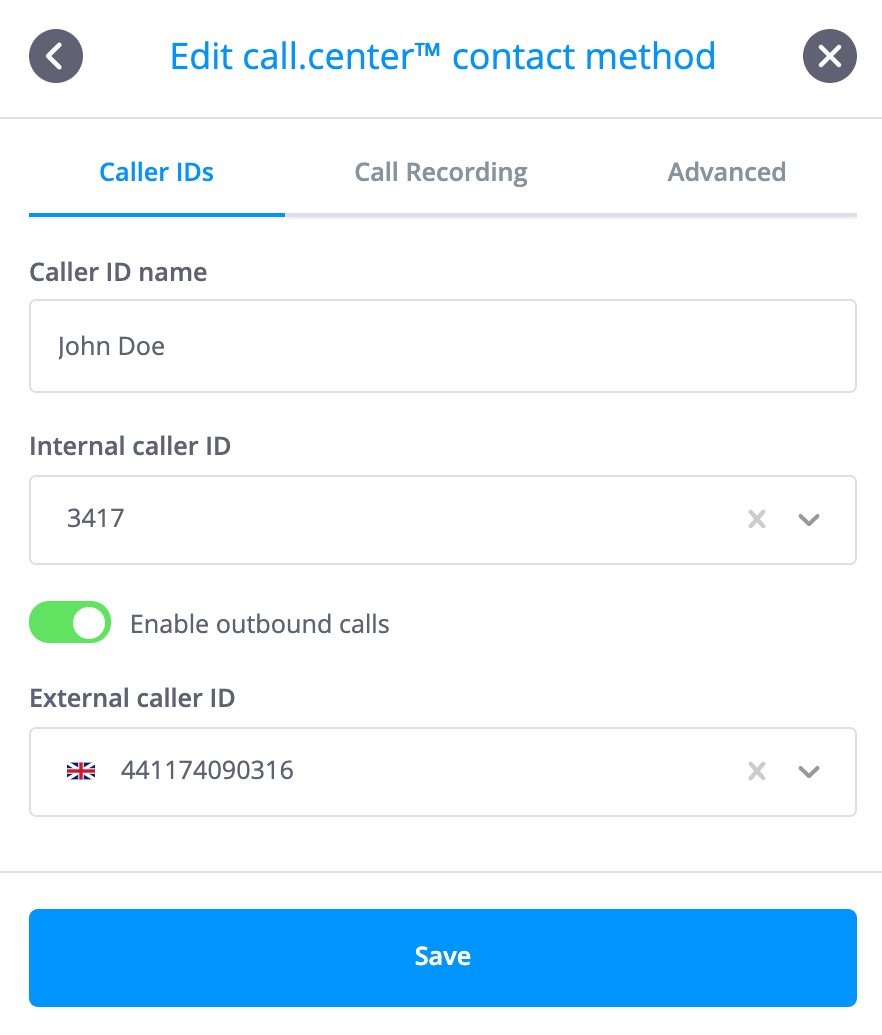The image depicts a webpage with the heading "Edit Call Center Trademark Contract Method." The layout is organized with a left-hand column shaded in blue, labeled "Caller IDs." Adjacent to this, there is a clickable section named "Call Recording" and a further option to the right tagged "Advanced."

In the main content of the page, the Caller ID name is displayed as "John Doe," while the Internal Caller ID is listed as "3417." A noticeable green button labeled "Enabled Outbound Calls" is situated prominently. 

Additionally, there is an indication of the External Caller ID, marked by a small British flag symbol, representing the Union Jack, alongside the number "441174090316." 

At the lower right, a blue-highlighted button reads "Save." The context suggests that the page might be a workspace interface or a record of call activities within a professional environment, possibly an employee's call log or settings.